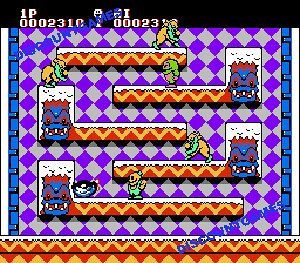The image is a screenshot from an old 1980s or 1990s side-scrolling game featuring pixelated, retro graphics. The scene is set against a dark and light purple checkerboard background, with a black strip at the top displaying the scores. The game consists of five platform levels, each colored in red with yellow zigzag patterns that resemble waves and seem to be coated with ice or snow. Scattered across these levels are various characters, including yellow ogres and other monsters. Prominently displayed at the end of each level is a dragon-like head, blue with red hair. Across the top-left to bottom-right corners in hard-to-read purple letters, the text "Discount Games" is faintly visible.